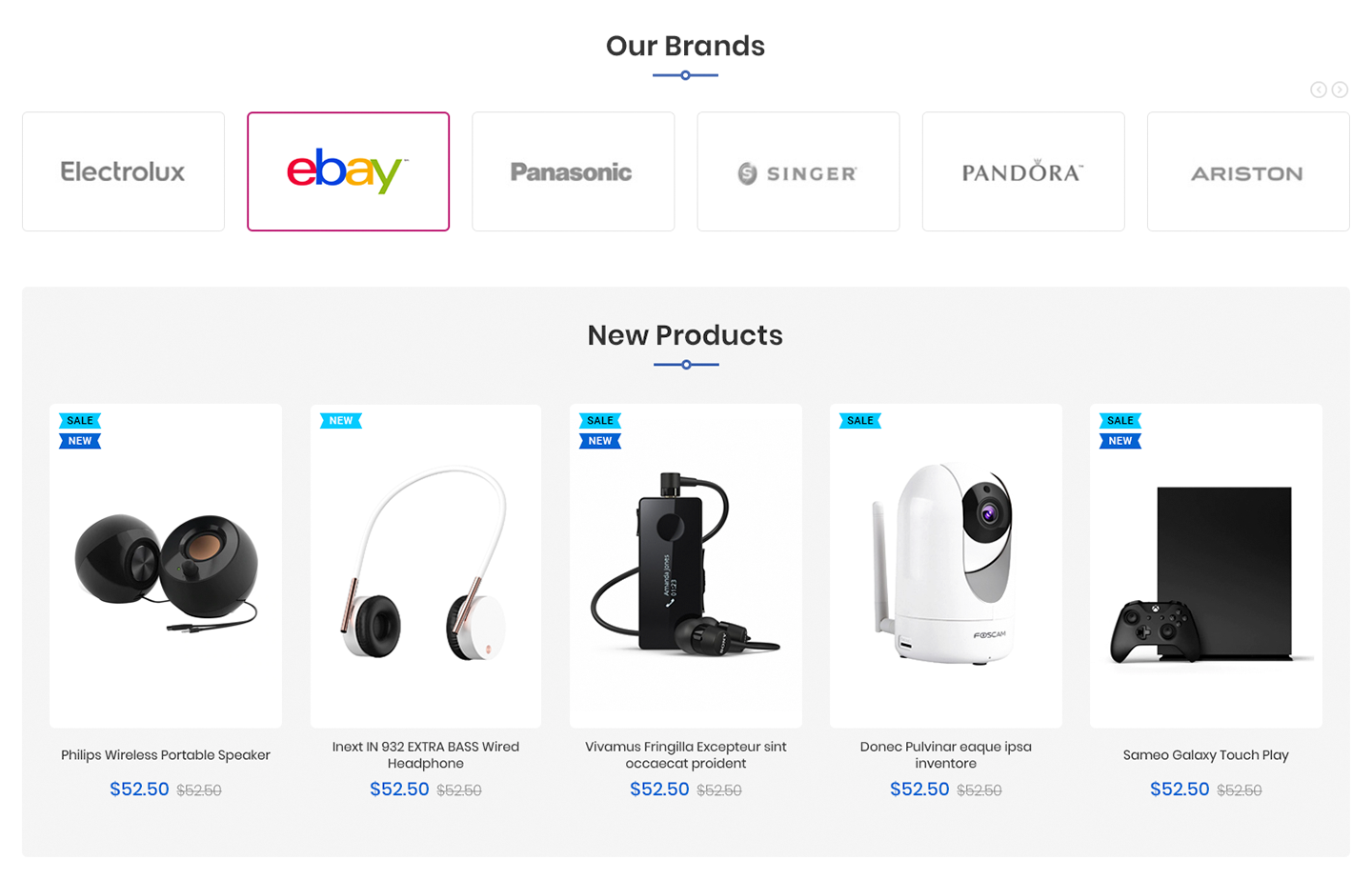This is a screenshot of a web page from "R Brands," featuring a clean, white background with a navigation bar at the top. The navigation bar includes six square icons arranged horizontally, each representing a different brand: Electrolux, eBay, Panasonic, Singer, Pandora, and Ariston. The eBay logo, which is colorful, is currently selected, while the other logos appear in gray.

Below the navigation bar is a section titled "New Products" situated within a light gray box. The title, centrally located at the top of the box, is underlined with a blue line that has a circle in the center. 

In this "New Products" section, there are five individual white boxes, each showcasing a different product:

1. **Philips Wireless Portable Speaker** 
   - Label: "Sale & New"
   - Product Image: Speakers
   - Price: $52.50

2. **Innext IN932 Extra Bass Wired Headphones** 
   - Label: "New"
   - Product Image: Headphones
   - Price: $52.50

3. **Vivimis Phryngelia Acceptor Synth Essentia Prontent**
   - Label: None specified
   - Product Image: Black box with a wire (description not in English)
   - Price: $52.50

4. **Donic Pulver Equae Ispa Inventor**
   - Label: None specified
   - Product Image: Possibly a webcam or security camera
   - Price: $52.50

5. **Samsung Galaxy Touch Play**
   - Label: None specified
   - Product Image: Gaming system
   - Price: $52.50